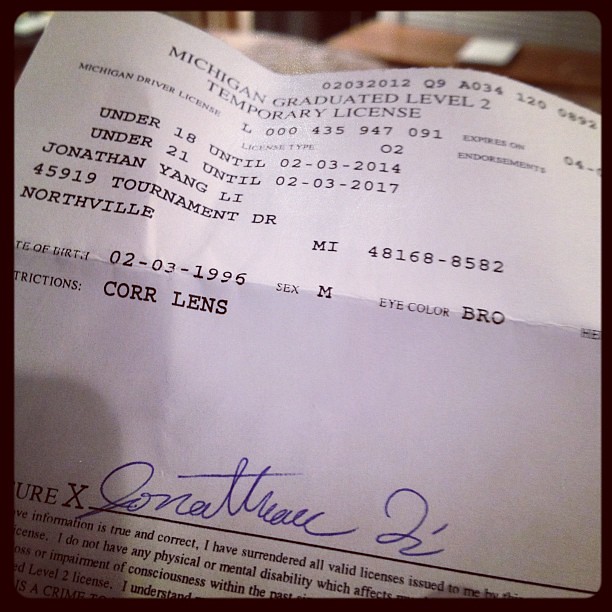This is a close-up photograph of a folded and then unfolded white piece of paper, which is a Michigan Graduated Level 2 Temporary License. The top of the document displays the license type in black capitalized letters. Immediately beneath, it reads "Michigan Driver License," followed by the actual license number: L000435947091. To the right of the license number, the expiration date begins with "04," but the rest is cut off by the right edge of the photo. Below this section, the document indicates "under 18 until 02-03-2014" and "under 21 until 02-03-2017."

The individual identified on the license is Jonathan Yang Lee, residing at 45919 Tournament Drive, Northville, Michigan, 48168-8582. His date of birth is 02-03-1996, making him a male with brown eyes who requires corrective lenses. The document includes his signature at the bottom, written in blue ballpoint pen, as "Jonathan Lee," along with a large "X" indicating where the signature should be placed. The paper has some creases, indicating it has been folded in half horizontally. The photograph shows additional black text below the signature area, partially cut off and too small to read clearly.